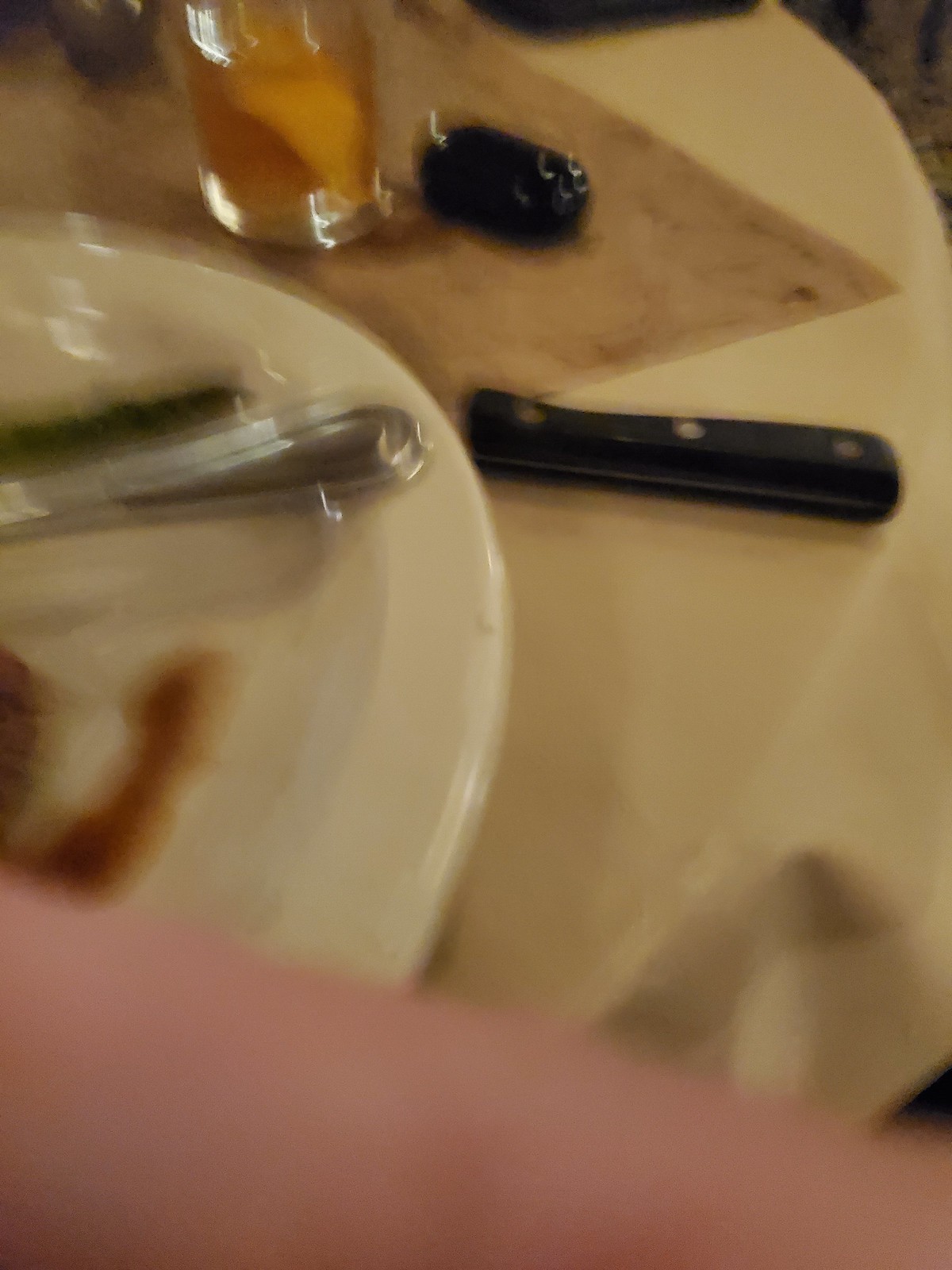In this slightly blurry image, a white dinner plate is prominently featured, placed on a round table covered with a white and tan tablecloth. The plate holds a serving of green vegetables, possibly asparagus, accompanied by a drizzle of brown sauce. A piece of silverware rests on the plate, and the wooden handle of a knife is visible beside it. In the foreground, the arm of a Caucasian individual partially obstructs the view, hinting at a candid and informal dining moment. In front of the plate, there is a drinking glass, which appears to contain a yellow lemon slice. Additionally, a small black object, possibly a condiment container or utensil, sits adjacent to the glass. The scene captures a moment of an inviting yet casual dining experience.